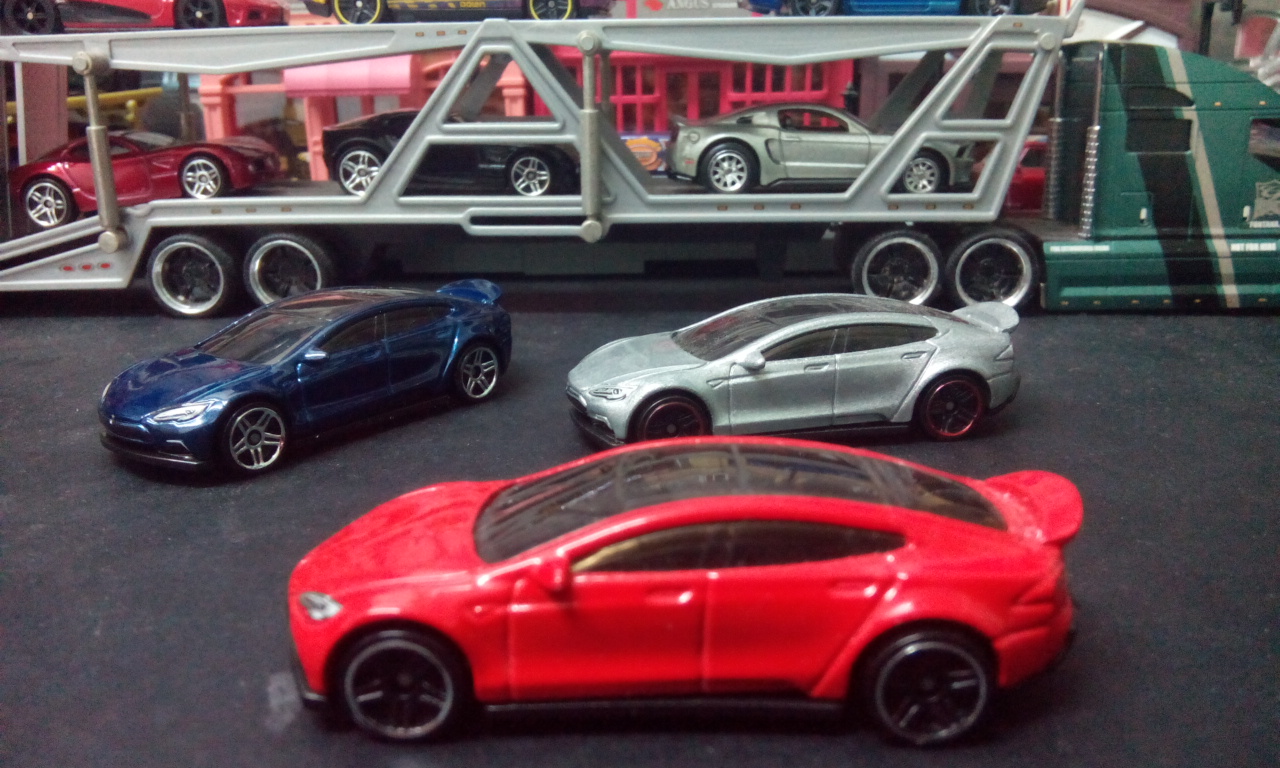The image is a horizontally oriented, color photograph capturing a collection of toy cars, likely Hot Wheels or Matchbox cars, arranged meticulously on what appears to be a black showroom-like floor. The foreground showcases three sports-style toy cars: a slightly blurred red car closest to the camera in the center, a blue car to the left, and a silver car to the right. These cars feature distinct details such as dark stripes across their tops, spoilers, and tinted windows, suggesting high-performance models. In the background, a green car hauler truck with a silver trailer and black and silver accents spans the image from left to right. This transport vehicle carries six additional toy cars: a red, black, and silver car on one level and another set of three that are harder to see clearly. The composition of the toys and their positioning hint at a miniature auto show display, highlighting the intricate details and vibrant colors of these model cars.